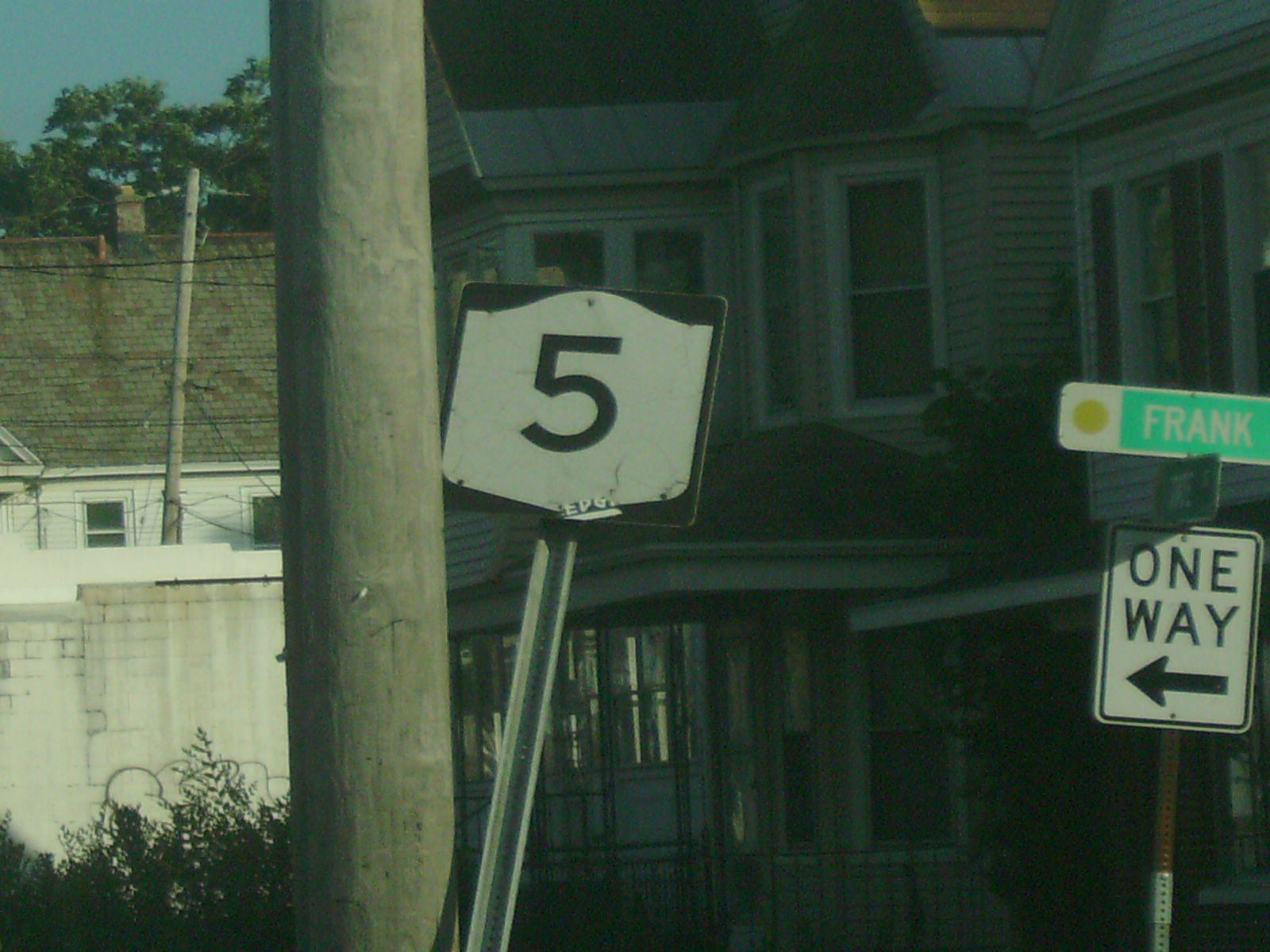In this outdoor image, the clear medium blue sky serves as a serene backdrop to a residential scene. Green treetops frame the upper portion of the image, transitioning down to a neighborhood of older homes. One prominent white house with a worn brown-grayish roof stands in disarray, showing age spots and dirt, while a larger gray house with a black roof is partially visible, both suggesting a state of neglect. Scattered throughout the scene, multiple telephone poles add a textured, gray aesthetic.

Central to the image, a metal sign on a single pole bears the number 5 in black text framed by a black border on a white background. This sign appears slightly tilted backwards and to the right. Nearby, another sign mounted on a pole prominently displays "One Way" with an arrow pointing left, rendered in white with black text and border. Adjacent to this, at a slight angle, are two perpendicular green street signs, one clearly marked "Frank," though the other sign is partially obscured.

Additional details suggest the photo may have been taken with a zoom lens or from within a car, enhancing its snapshot character and adding an interesting perspective, perhaps accentuated by post-processing filters. Despite the photogenic sky, the overall ambiance conveys a sense of aged charm and quiet neglect in this typical residential street scene.